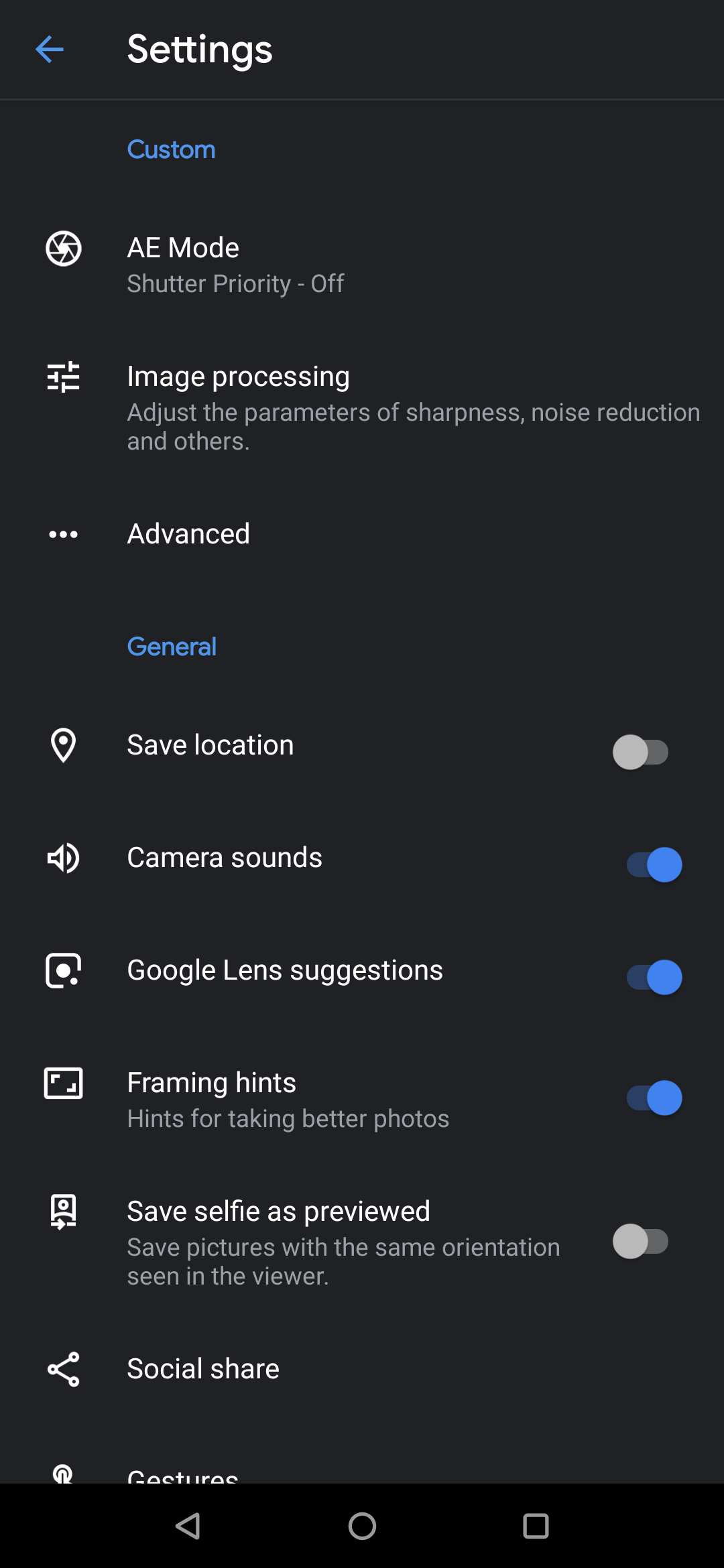The image displays a settings menu on an Android device in night mode, evidenced by its all-black background. The screen is clearly an Android interface, identifiable by the three classic navigation buttons at the bottom—back, home, and recent apps.

At the top of the menu, the word "Settings" is prominently displayed. Below it, the menu is divided into several sections:

1. **Custom** - This section contains configurable options for the user to personalize their experience.
   
2. **AE Mode** - Shutter priority is turned off, indicating that the auto-exposure settings are being used without any manual shutter speed adjustments.

3. **Image Processing** - This section provides parameters for adjusting sharpness, noise reduction, and other image enhancements, aimed at refining the photo output.

4. **Advanced** and **General** - These broader categories likely contain additional specific settings.

5. **Safe Location** - Toggled off, implying location data for photos will not be saved.
   
6. **Camera Sounds** - Toggled on, enabling sound feedback when taking pictures.

7. **Google Lens Suggestions** - Toggled on, allowing the Google Lens to suggest information and actions based on the camera’s view.

8. **Framing Hints** - This likely provides guidance on how to frame subjects in photos if enabled.

9. **Save Selfie As Previewed** - Toggled off, meaning selfies will not be saved as they appear on the preview screen.

10. **Social Share** - An option that probably allows for easy sharing of photos to social media platforms.

11. **Gestures** - A button located at the bottom, possibly providing options for gesture-based controls within the camera app.

On the left side of the screen, there are several icons representing different functions such as location, sound, and framing, giving quick access to these features.

In summary, the screenshot captures the camera settings menu of an Android device, laid out in a detailed and organized fashion, primarily focusing on various camera configuration options.